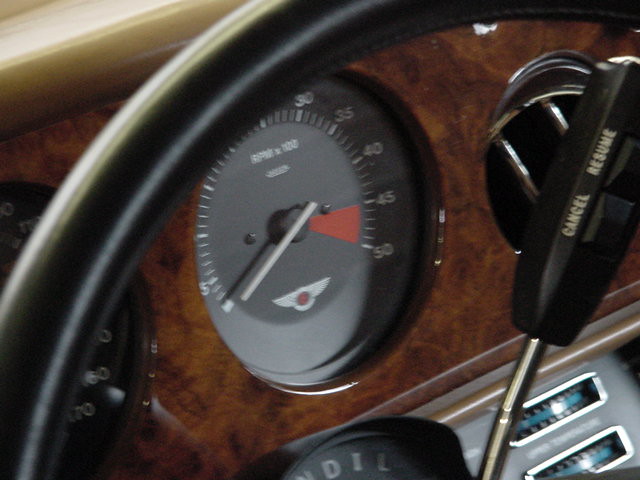This image showcases a detailed view of a car's dashboard, captured with remarkable clarity. Dominating the upper portion of the frame is a large, circular black shape. On the right side, there's a metallic component that resembles a screwdriver, featuring a small circular black piece at its tip. This component includes two buttons labeled "Cancel" and "Resume."

In the background, the dashboard reveals itself with a rich brown hue, punctuated by multiple circular openings. On the right, there's a glass-covered circular opening with a black background, and centrally another circular opening with a gray face. The gray circular opening prominently displays numeric increments: 30, 35, 40, 45, and 50. Between the 40, 45, and 50 markers, there’s a section highlighted in red, with a metallic pin pointing towards these numbers.

Flanking the lower part of the image, blueish bars hint at additional dashboard features. This intricate scene encapsulates the various elements of a luxurious car's steering wheel area, showcasing the fusion of functionality and design.